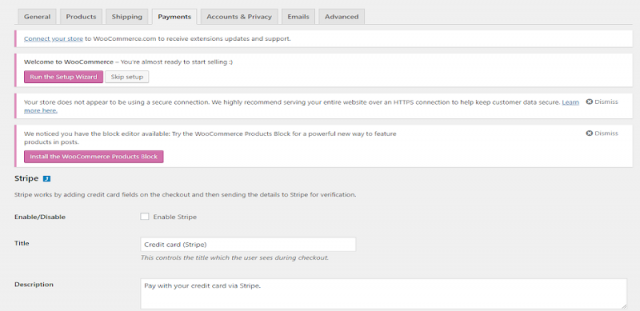This screenshot showcases a desktop user interface of a complex, business-oriented software application or website. The layout is industrial and utilitarian, suggesting functionality over aesthetic appeal. The interface is populated with numerous clickable buttons, text fields, sections, categories, and tabs, indicative of a sophisticated suite of tools designed for business use rather than general consumer purposes.

The primary focus is the "Payments" tab, among several others such as "General," "Products," "Shipping," "Accounts and Privacy," "Emails," and "Advanced." In this tab, various control options are presented, including buttons labeled "Run the Setup Wizard" and "Skip Setup." Additionally, there is an option to install a "Products Block."

The "Payments" section specifically features options like "Enable" and "Disable," and includes support for integration with Stripe, a well-known payment processing service. Users can also input a title and description, adding to the customizable settings within this section. The overall interface suggests that this software is built to manage intricate business operations and requires a certain level of expertise to navigate effectively.